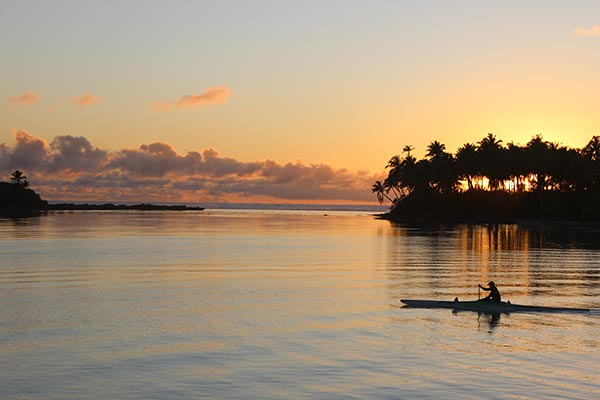The photograph captures a serene sunset scene over a calm body of water, which looks like a lake. The sky transitions from a very light blue at the top to vibrant hues of orange, pink, and yellow as it nears the horizon. Low-lying clouds scatter across the sky, adding texture to the backdrop. The scene is mirrored on the water's surface, casting shimmering reflections of the sunset's warm colors.

On the right side of the image, there are silhouettes of palm trees and an island, while additional trees are faintly visible on the left side, suggesting a continuation of the landscape. In the bottom right corner, a solitary individual is seen kayaking, their black outline and the kayak clearly defined against the twilight water. The golden hour lighting, combined with the calmness of the water, creates a tranquil and picturesque setting.